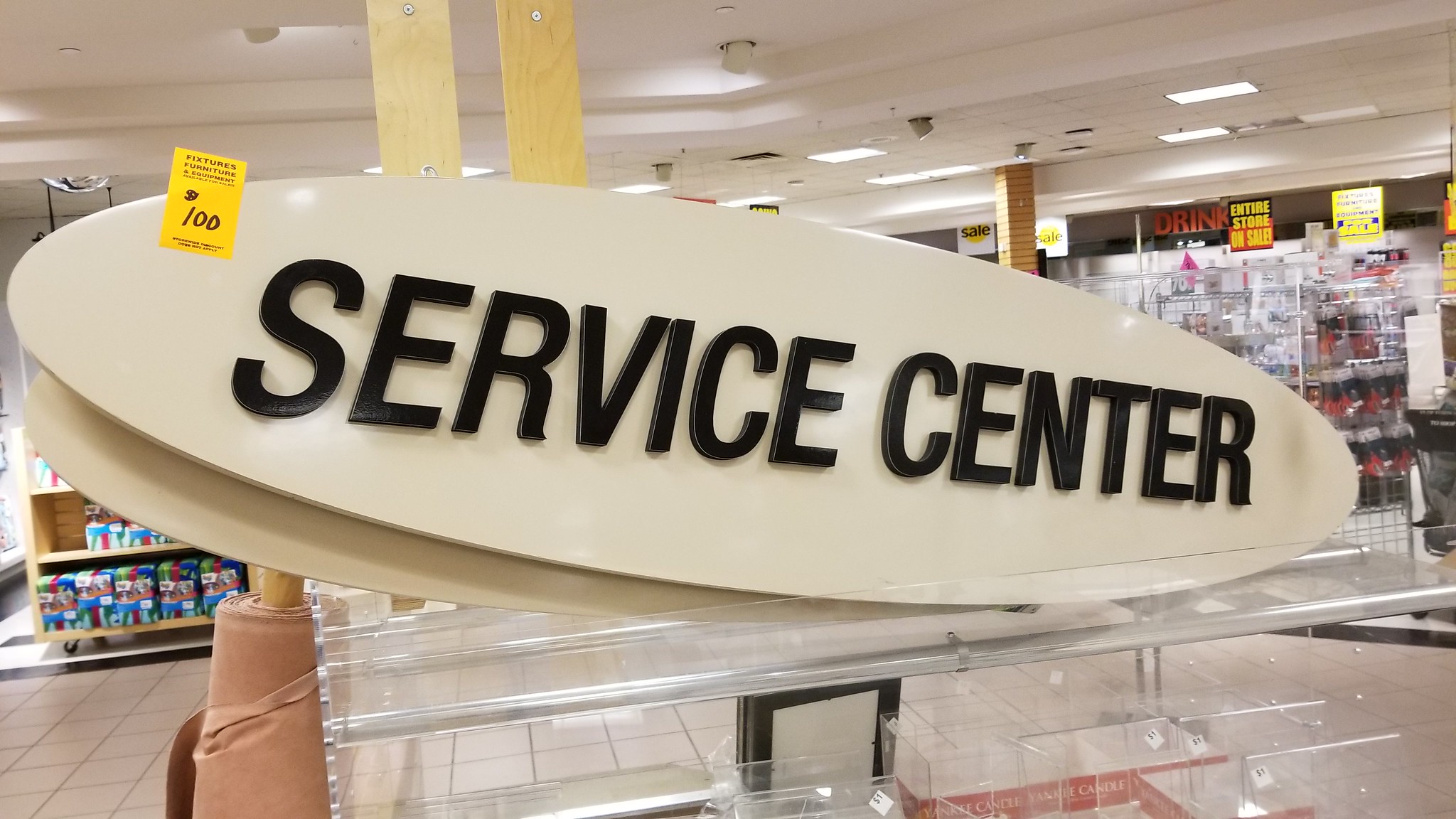The image depicts the interior of a retail store, with the focal point being a large, oval-shaped beige sign prominently displaying "Service Center" in bold black letters. Attached to this sign is a yellow sticky note marked with "100," suggesting it might be part of a liquidation sale. The sign is mounted on a white stand, which features clear shelves and a support on the left. Surrounding the sign are silver and white shelving units lined with various items. The background reveals more shelving with distinct signage, including a red "Drinks" sign above drink shelves and a wooden shelf on the left stocked with packaged snacks in blue and red boxes. The store is illuminated by a combination of beige spotlights and rectangular fluorescent lights on the white ceiling. Partitions and additional signs create a sense of depth within the space.